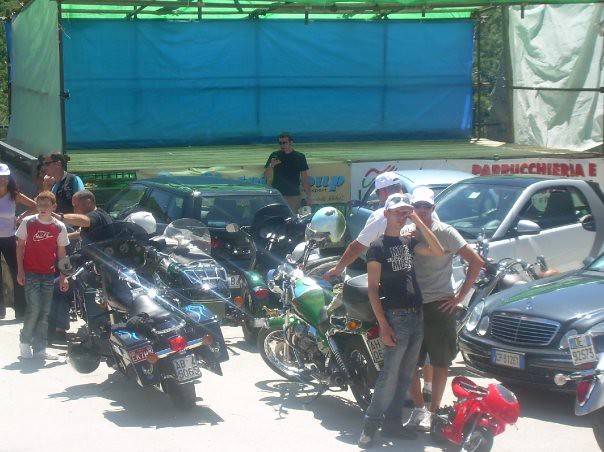The photograph captures a lively outdoor event, possibly a rally or festival, set in a parking lot under the bright midday sun. At the top, the background reveals a temporary stage partially covered by green and blue tarps, supported by silver aluminum pipes. The stage's light green wooden platform is adorned with several obscured posters in a foreign language. Surrounding the stage area are multiple motorcycles and cars, including a green motorcycle, and a distinctive Mercedes Benz with European license plates.

The chrome on the motorcycles shines brightly, amplified by the sunlight, creating noticeable lens flares. In the bottom right corner, a group of three men, dressed for warm weather and wearing white hats, stands engaged with each other. To the left, another small group includes a child in a red Nike shirt and green jeans, a lady in a white tank top and black pants with her hands on her hips, and a few others mingling near the parked vehicles.

People are scattered throughout, with some walking into the area and others absorbed in conversations. A notable figure near the stage is a man in a black t-shirt and sunglasses, possibly on his phone. The atmosphere suggests a casual yet organized gathering, bustling with interactions and activities centered around the stage and the impressive lineup of vehicles.